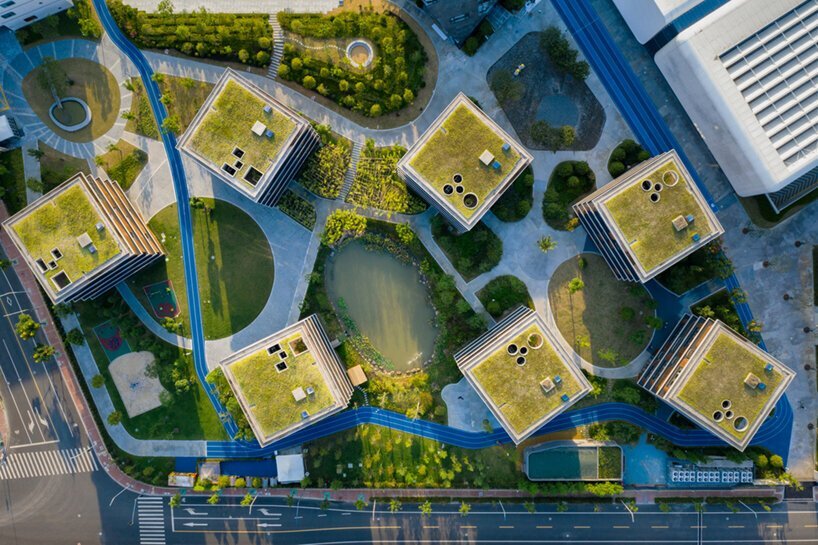This horizontal rectangular color image appears to be an aerial view, possibly computer-generated or photographed, offering a detailed look at an urban park area. The scene comprises seven square buildings of about five stories each, organized in two distinct layers—four at the top and three below, all slightly tilted at different angles. Each building features grassy rooftops, blending seamlessly with the surrounding lush, well-manicured greenery, and is adorned with various shapes that resemble air conditioning units or similar structures. Interspersed among these buildings are walkways and sidewalks, facilitating easy movement throughout the park area. In the foreground, a paved road with a yellow dashed line in the middle and white lines on the periphery runs horizontally across the image from the far left to the far right. This road intersects with another vertically oriented street on the left side, complete with crosswalks and directional arrows. Adding to the picturesque scene is a small pond, enhancing the natural aesthetics of the entire landscape.